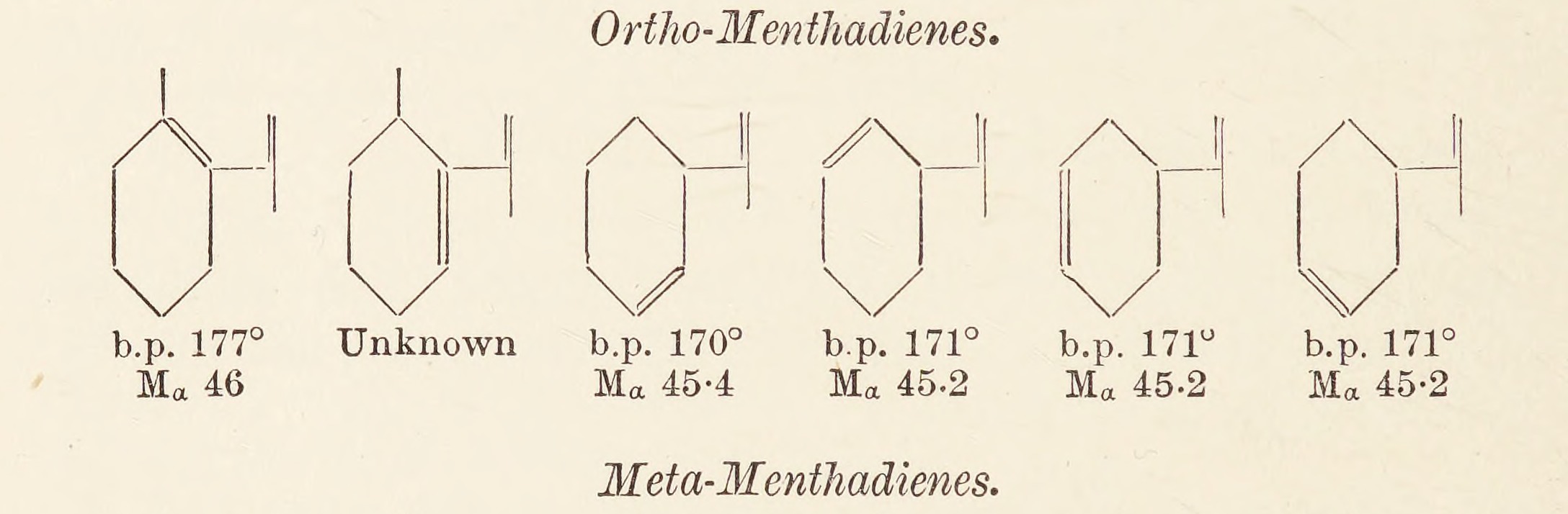The image is a scientific chart that seems to be a page from an old chemistry textbook or an educational poster. It has a rectangular shape and the background is a faded tannish or off-white color, giving it an aged look. The chart displays text at the top and bottom, with a series of hexagons aligned horizontally across the center. Each hexagon is accompanied by specific text underneath.

At the very top of the image, the title reads "Ortho-Menthadienes," and at the very bottom, it says "Meta-Menthadienes." Starting from the left, the first hexagon has text below it that reads "BP 177° MA 46." The hexagon next to it has "unknown" written underneath, followed by a third hexagon labeled "BP 170° MA 454." There are several more hexagons following this sequence, each with similar annotations.

The overall appearance and style suggest this chart is likely used for educational purposes, specifically within the context of chemistry, contrasting pale background hues with black text and hand-drawn illustrations.